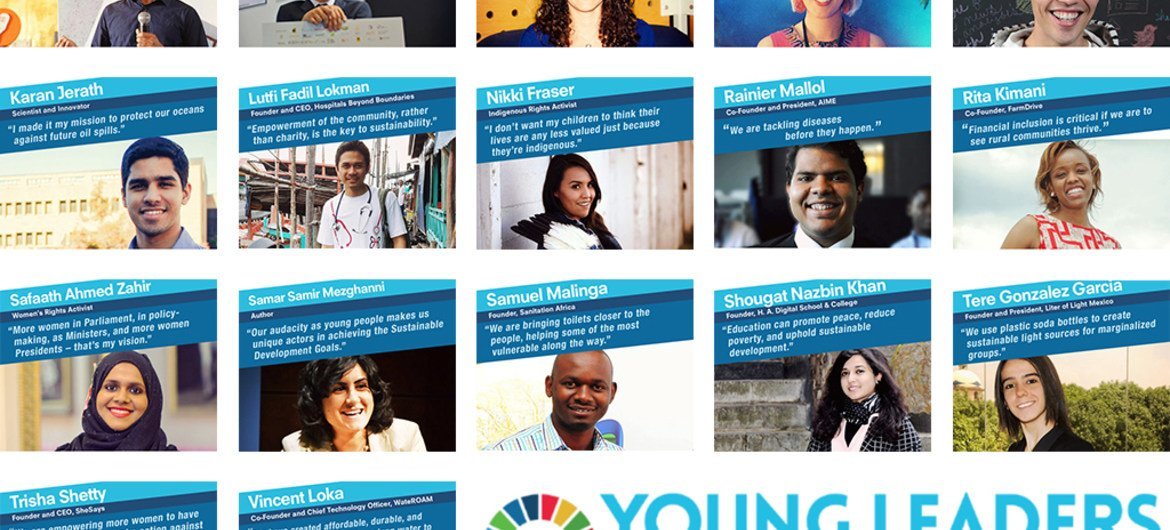The image is a collage consisting of multiple sections, primarily depicting young leaders accompanied by their quotes and names. At the top, part of the image is cut off, making it hard to discern specific details or people. 

Below the cutoff, there are two full rows, each containing five columns. The sequence of backgrounds and text colors varies as follows: it begins with a white section on the upper left, transitions to a baby blue section with white text providing the person's name, followed by a deep purple section, and then a darker blue section featuring a quote from the individual along with their photograph.

Among the individuals featured are:
- **Carden Jareth:** Appears to be of Indian descent.
- **Lucy [last name not visible]:** Additionally, an Indian-looking individual.
- **Nikki Frazier:** Described as an Indian-looking woman.
- **Ranier Mello:** Another individual of Indian ethnicity.
- **Rita Kimia:** Likely Black, based on the description.
- **[Name not provided]:** Described as Muslim or Arabic.
- **Samir [last name not visible]:** Likely of Arabic descent.
- **Samuel [last name not visible]:** Described as a very dark-skinned Black individual.
- **[Something] Khan:** Indicated to be Arabic.
- **Tara Gomez/Gonzalez/Garcia:** Likely Hispanic.

Each person has a corresponding quote displayed beside their images. Additionally, there are two further individuals at the bottom of the image, whose details are not discernible.

On the right-hand side of the collage, set against a white background, there is a blue text that reads "Young Leaders."